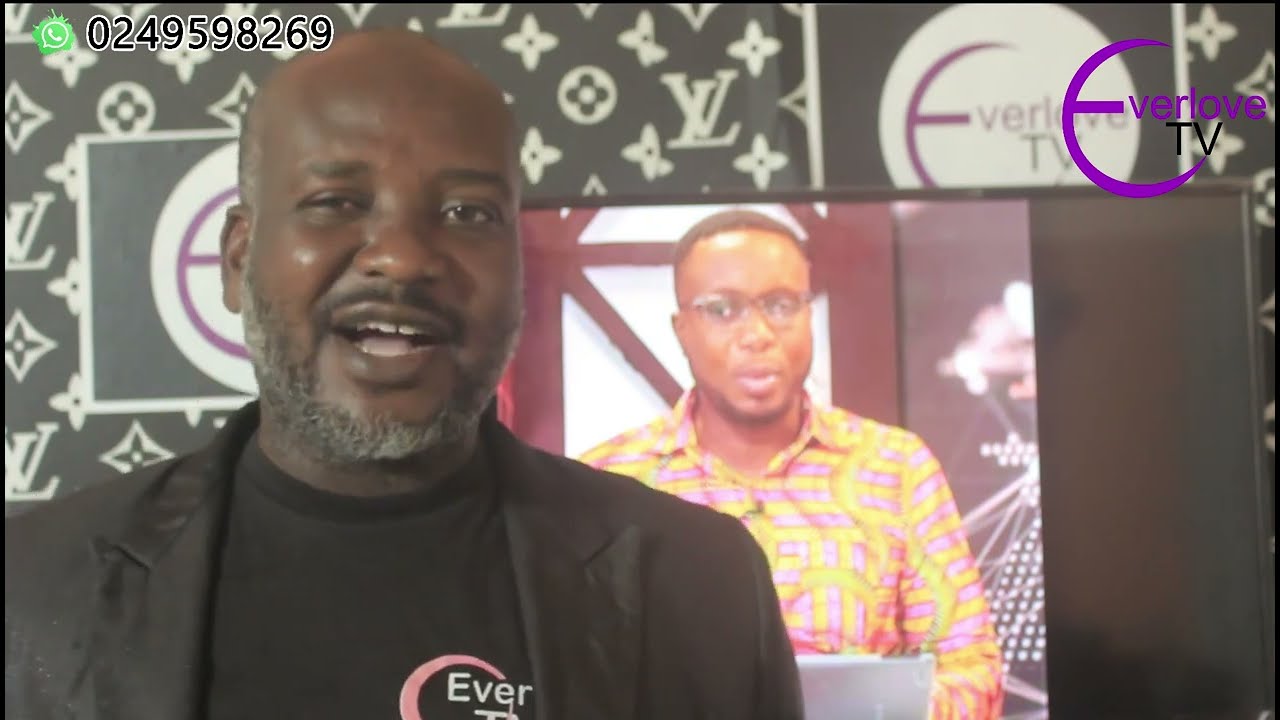This image is a screen grab from a TV show or video stream named "Everlove TV." Dominating the left half of the picture is an African-American male with a gray beard and mustache, a shaved head, dressed in a black sport coat over a black t-shirt featuring a pink and white Everlove TV logo. The background exhibits a black and white diamond and circle pattern reminiscent of a designer brand, decorated with multiple iterations of the Everlove TV logo. To the upper right, a purple and black circular emblem prominently displays the large, curved 'E' of Everlove TV. In the foreground, a green telephone with the number 024-959-8269 is visible. Behind the main speaker, a TV screen shows another man wearing glasses and a yellow button-down shirt with pink lines, set against a red and white stage. This secondary figure appears to be on a different stream or part of the show, contributing to the overall dynamic of the broadcast.